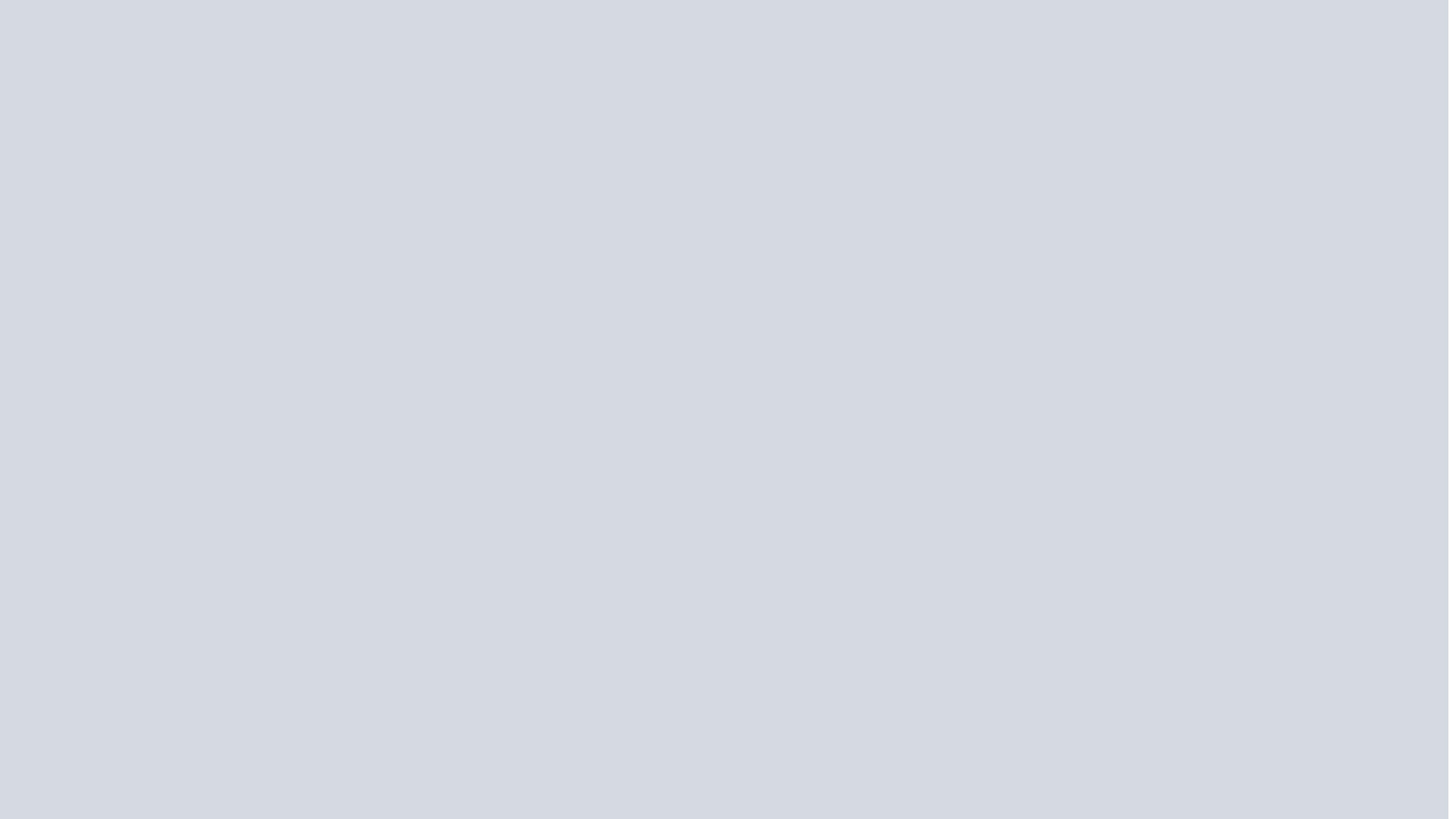The image depicts a uniformly light gray background without any objects, text, or stylistic elements. The entire screen is filled with a consistent shade of light gray, devoid of gradients or variations in color. The tone is a soft mix between dark gray and white, resulting in a subtle, neutral gray hue. The image appears featureless and plain, making it unclear whether it is a blank canvas, an unloaded image, or simply a minimalist design.